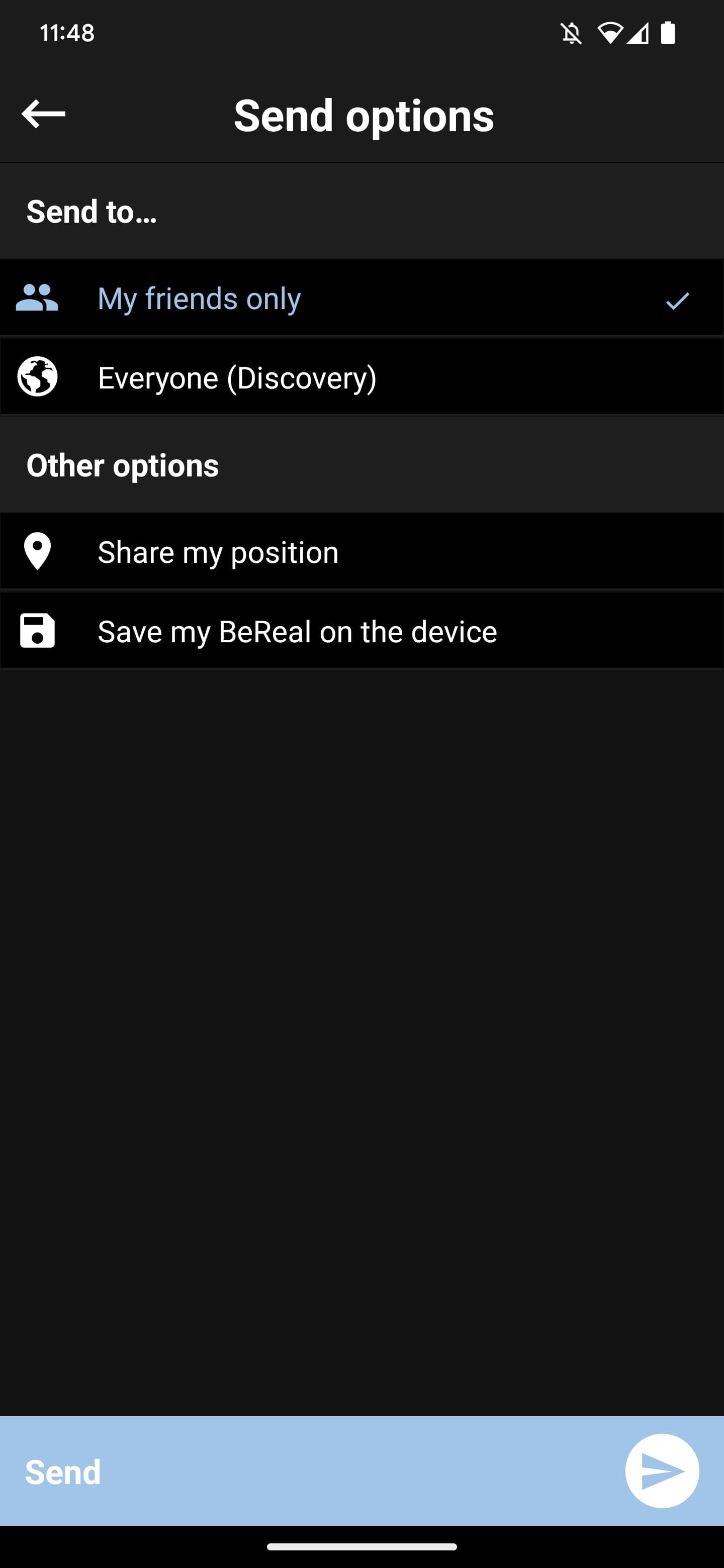The screenshot depicts a very dark gray interface with predominantly white text, designed for selecting send options. At the top of the screen, the title "Send Options" is displayed, accompanied by an arrow pointing left. Directly below, the label "Send to" appears, followed by "My Friends Only" in blue font, with a checkmark beside it. Underneath, the option "Everyone" is listed, accompanied by "Discovery" in parentheses. 

Further down, in the same dark gray background, the category "Other Options" is introduced. Resuming the white text on a dark background, two options are presented: "Share My Position" and "Save My BeReal on the Device."

At the very bottom of the screen, there is a sky blue bar with the word "Send" in white letters, next to a white arrow enclosed in a circle. Immediately below this bar is a small thin white line and a tiny black bar, providing a subtle visual divider to the bottom edge of the interface.